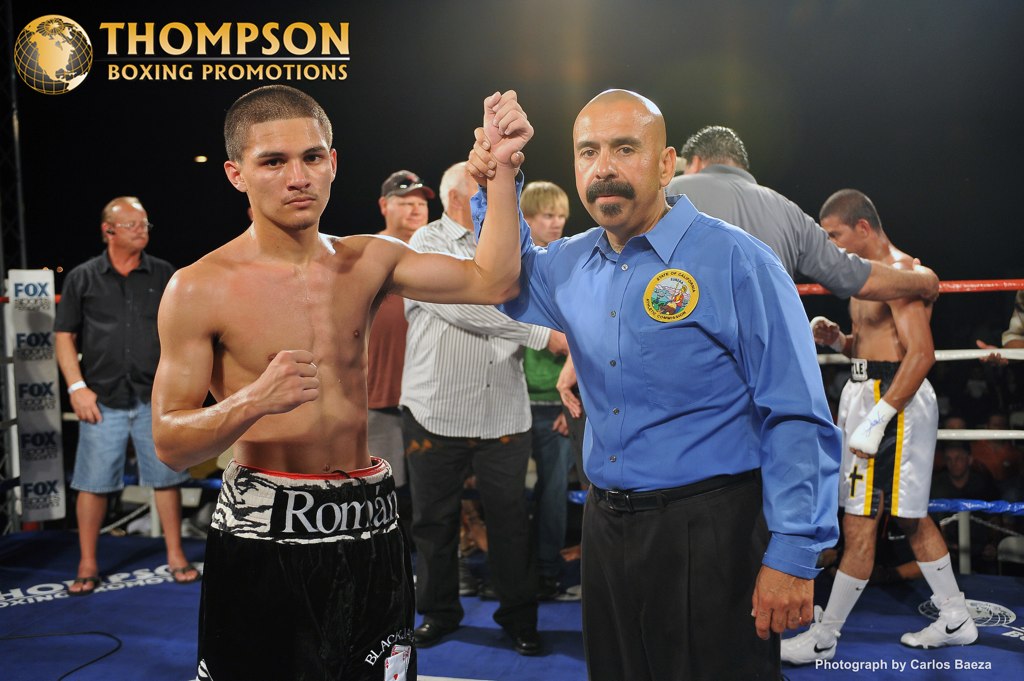The photograph captures a victorious moment inside a boxing ring, prominently displaying a shirtless Latino boxer on the left, wearing black shorts with 'Roman' inscribed around the waistband. His right fist is triumphantly raised in the air, while his left arm is elevated by his coach, also of Latino descent, signifying his victory. The coach, dressed in a blue button-down shirt with black pants, has a tanned complexion and a completely shaved head with a moustache. In the top left corner of the image, the emblem of a globe with gold land and a black grid ocean appears, accompanied by the text 'Thompson Boxing Promotions' in gold. Behind the central figures, other men can be seen inside the ring, surrounding the losing fighter, who is similarly shirtless and wearing white, black, and yellow shorts. The ring floor is blue, and the entire background is dark, emphasizing the dramatic moment. The bottom right corner of the image bears the inscription in white text, 'Photographed by Carlos Beza.'